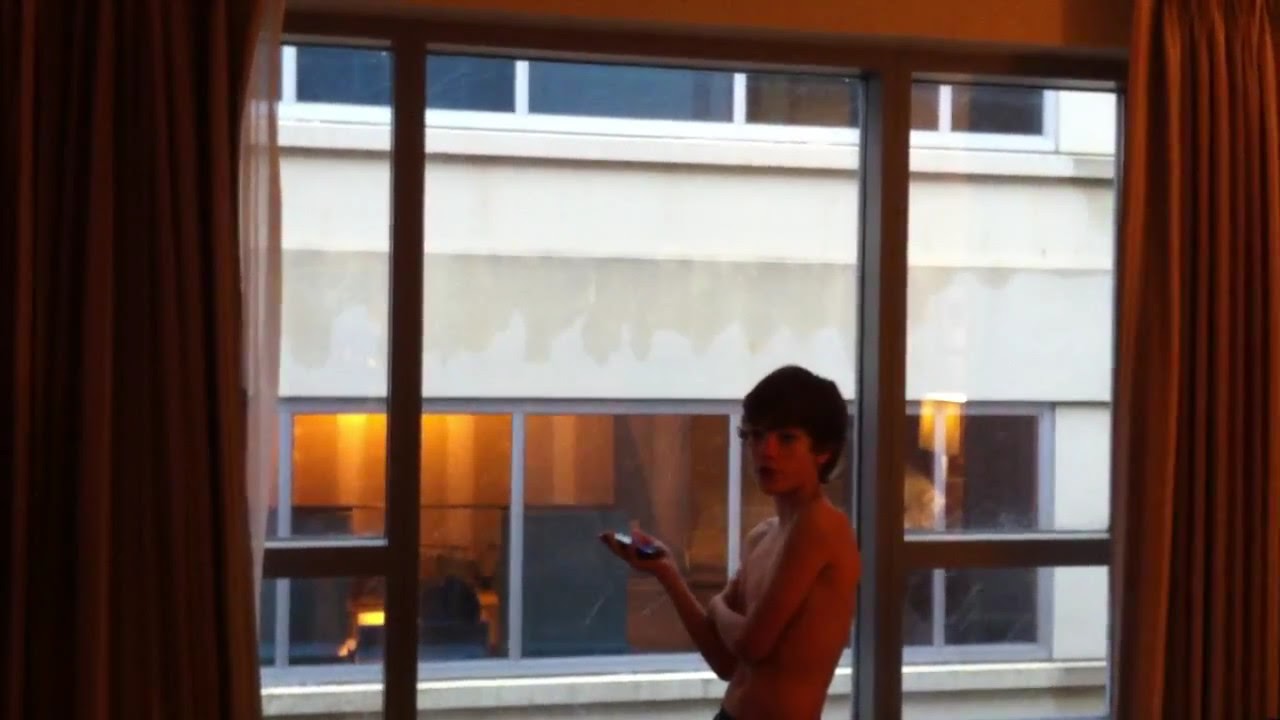The image portrays a color photograph of a young Caucasian boy, likely between 10 to 13 years old, standing shirtless in front of an open window in a room, possibly in a high-rise building or apartment complex. The boy has short brown hair, is relatively skinny, and holds a cell phone in his right hand while his left arm is crossed over his chest. He is wearing dark-colored shorts. The composition is in landscape orientation, with the boy positioned near the bottom of the frame, turning slightly to look over his shoulder towards the viewer. The window behind him has burgundy or reddish-orange curtains pulled to the sides, revealing another sheer white curtain behind them. Through the window, another building with similar concrete structure and rows of windows is visible, alongside a beige stucco section. The photograph, characterized by representational realism, focuses on both the boy and the urban scenery outside.